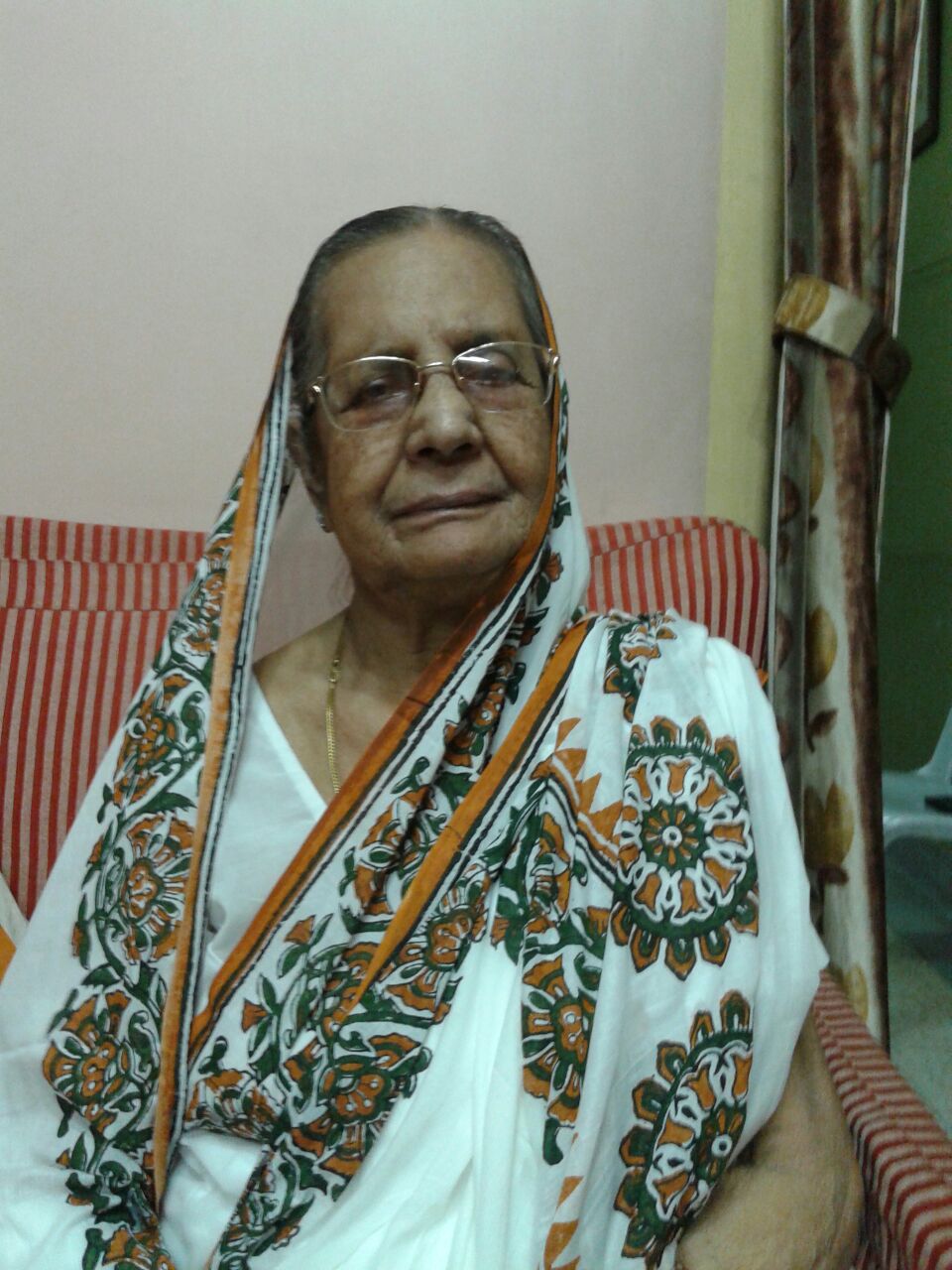This is a detailed photograph of an elderly woman, likely in her 70s or 80s and of possibly Indian or Pakistani heritage, sitting on a red and gray-striped couch. She has short gray hair, neatly combed with a part on the left side toward the center, and is wearing wire-rimmed glasses. Her skin is brownish, indicative of her ethnic background, and she has visibly aged with the passage of time. Draped in a traditional sari, white with a flowing and thin cotton texture, the garment is adorned with a floral pattern in green and orange hues. Around her neck, she wears a gold necklace adding a touch of elegance. The ambiance behind her features a white wall, a curtained doorway with a green and brown satin-like curtain on her left, and a light-colored floor visible in the background. Her expression is a mix of emotions; while one description suggests she is smiling and content, another implies she appears sad, possibly having cried recently. Overall, the image captures a complex blend of grace and life experiences.